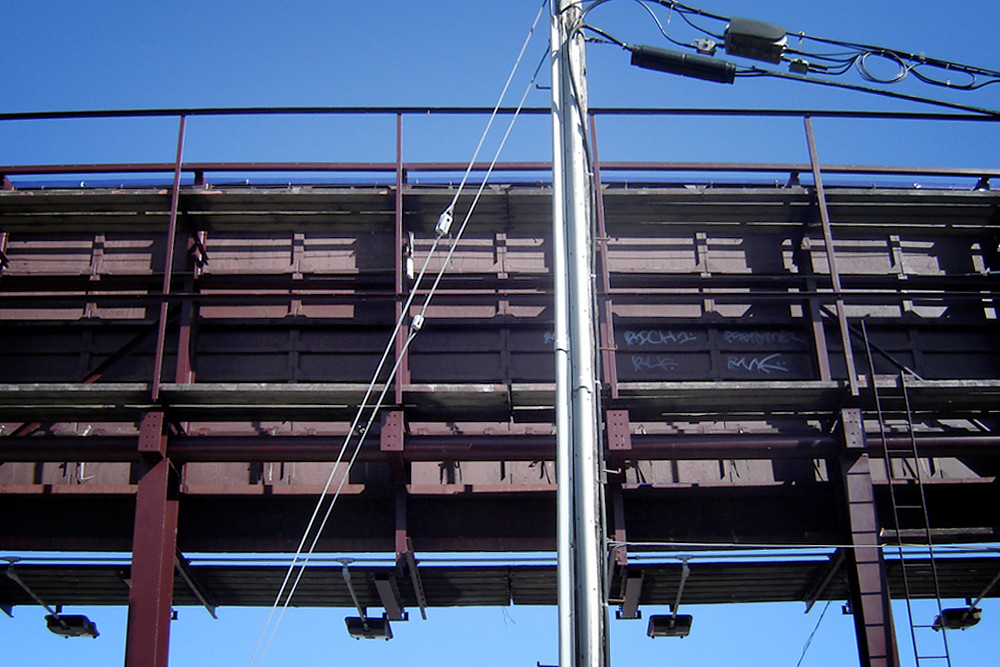The image showcases the back of a billboard, intricately supported and wired. Dominated by metal brackets running vertically and horizontally for structural integrity, the billboard features four square lights projecting from the bottom edge. A central silver pole stands out, connected by two hefty cables that run downwards to the base of the billboard. To the right, two black cables extend from the pole, each adorned with a black box. Smaller, zigzagging cables intricately weave along these rightward cables, adding to the complexity. The entire structure is upheld by two primary supports that boast a dark maroon, rust-like hue, complemented by smaller supporting elements of the same color. A metal ladder is positioned at the bottom right, with rungs enclosed between two vertical lines. This scene unfolds under a clear, blue sky devoid of clouds and sunlight.